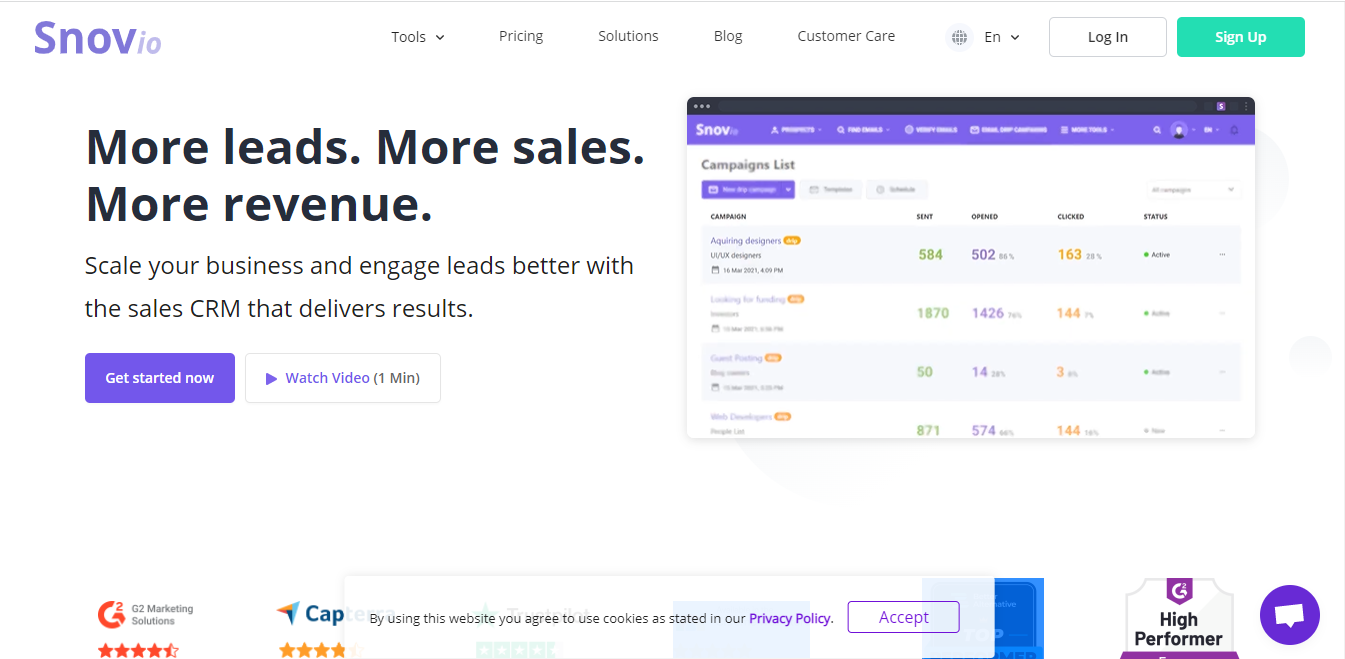Screenshot of the snove.io Website Homepage

The homepage of snove.io, a dynamic sales platform designed to help businesses scale and engage leads more effectively, is vividly presented. The main headline boldly states, "More Leads, More Sales, More Revenue," encapsulating the core benefits of the platform. Beneath it, a compelling subtitle reads, "Scale your business and engage leads with the sales CRM that delivers results."

Central to the page, an eye-catching "Get Started Now" call-to-action button in a striking purple box invites users to begin their journey. Adjacent to it, a lighter-colored button labeled "Watch Video One Minute" entices visitors to learn more through a brief visual overview. An informative illustration of a campaign list dashboard showcases the platform’s clean and intuitive interface, highlighting key metrics such as campaigns, sent emails, opened emails, clicked emails, and campaign statuses.

The top navigation bar is neatly organized with links to essential sections: Tools, Pricing, Solutions, Blog, and Customer Care. It also features options for logging in, signing up, and selecting the preferred language.

At the bottom of the page, the credibility of snove.io is reinforced with logos and ratings from renowned review platforms such as G2 Marketing Solutions and Capterra, accompanied by positive testimonials praising the service. A cookie consent notice is subtly positioned at the bottom right corner, complete with an "Accept" button. Enhancing the site’s authority and usability, a high performer badge and a help messenger icon are unobtrusively set at the far right bottom corner of the page.